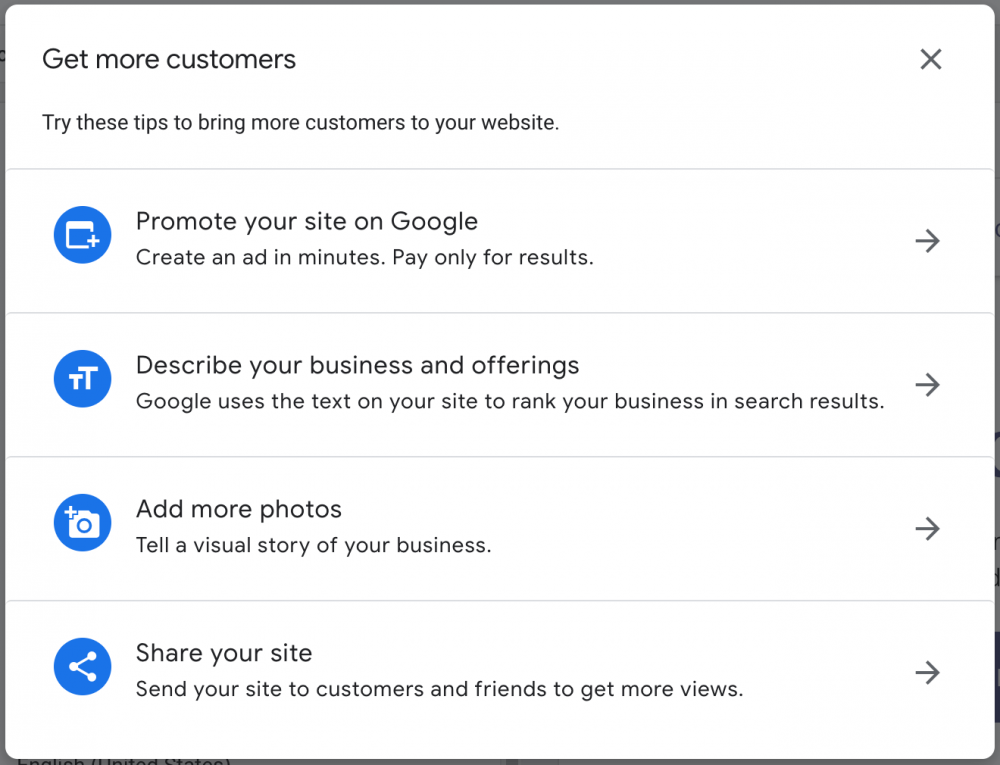This image is a detailed screenshot of a section of a Google-branded website focused on assisting users with selling and advertising through Google's platform. The top of the page features a headline in bold, urging users to "Get More Customers" and offers various strategies to drive more traffic to their website.

Below the headline, there is a small blue icon depicting a stylized web browser outline with a plus sign. Adjacent to the icon, text encourages users to "Promote your site on Google: create an ad in minutes, pay only for results," with an actionable button to initiate the ad creation process.

The following tip is represented by an icon with two uppercase "T"s of differing sizes, signifying text. The accompanying text advises users to "Describe your business and offering. Google uses the text on your site to rank your business in search results," with another clickable option for further details.

Continuing, there is an icon of a camera with a plus sign next to it. The tip here reads "Add more photos: tell a visual story of your business," with a link provided for users to explore additional guidance on adding visuals.

Lastly, an icon depicting the classic share symbol, shaped like a "V" with three dots at its points, introduces the tip "Share your site: send your site to customers and friends to get more views." This also includes a link for users to gain more information.

Each tip offers actionable buttons to learn more or proceed, making the interface both informative and interactive.